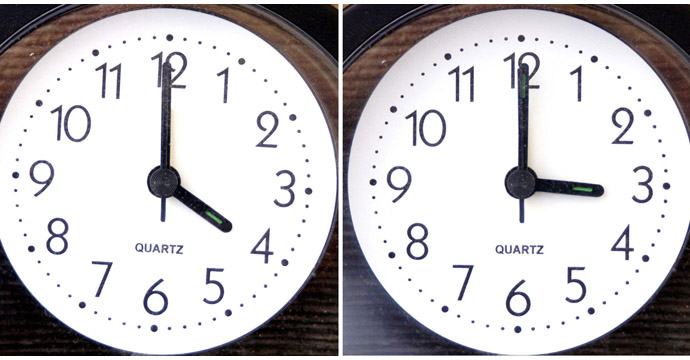The image depicts two side-by-side photographs separated by a vertical white line, each featuring the same analog clock set to different times. The clock has a distinctive dark wood textured border and a round face that is primarily white. Black numerals from 1 to 12 encircle the face, complemented by larger black dots marking each hour and smaller black dots signifying the minutes in between. Both black minute and hour hands are present, with the hour hand distinguished by a small green line. The brand name "QUARTZ" appears in capital letters beneath the hands. The left clock displays the time as 4 o'clock, while the one on the right shows 3 o'clock.